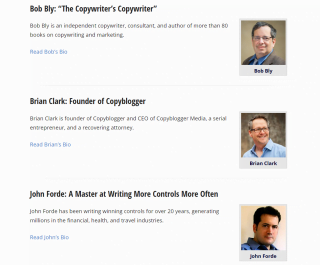The image appears to be a detailed segment from a copywriter's blog, featuring a highly visual and descriptive layout. The square image has a very pale gray, almost white background. On the right side of the image are three headshot photos aligned vertically in squares. Each photo has the respective person's name displayed below it.

- **Top photo:** Labelled **Bob Bly**. Bob Bly is a middle-aged man wearing glasses.
- **Second photo:** Labelled **Brian Clark**. Brian Clark is also a middle-aged man wearing glasses.
- **Third photo:** Labelled **John Forde**. John Forde is a younger man with black hair and is not wearing glasses.

To the left of these headshots, there are small blurbs that give more context about each individual. The names and titles are in bold, followed by their descriptions.

- **Bob Bly:** 
  - Title: "The Copywriter's Copywriter."
  - Description: "Bob Bly is an independent copywriter, consultant, and author of more than [unreadable number] books on copywriting and marketing." 
  - Link: There is a clickable link to "Read Bob's Bio."

- **Brian Clark:**
  - Title: "Founder of Copyblogger."
  - Description: A brief sentence about him and his achievements.
  - Button: A clickable button to "Read his bio."

- **John Forde:**
  - Title: "A master at writing more controls more often."
  - Description: A brief sentence about his expertise.
  - Button: A clickable button to "Read his bio."

The concise yet informative structure of the text combined with the visual presentation of headshots and clear labels creates an organized and professional layout, making it easy for readers to identify and learn more about each featured copywriter through the provided links.